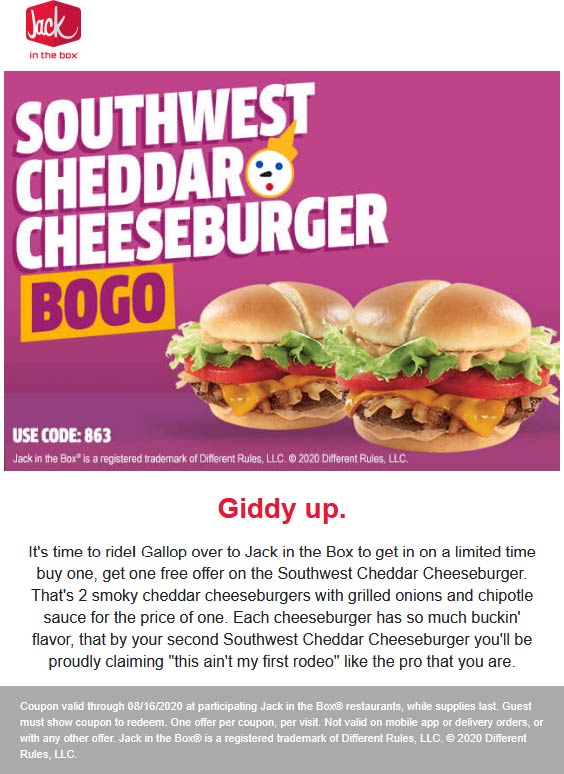**Caption:**

A promotional message from Jack in the Box is displayed. In the upper left-hand corner, there's a red logo featuring two sides of a cube with the word "Jack" in white cursive letters (capital "J" and lowercase for the rest), and "in the box" written in red underneath in small font.

Dominating the image is a vibrant square section with a purplish background. Large white text announces the "Southwest Cheddar Cheeseburger." An icon of Jack in the Box's head—a circle with two blue circular eyes, a small black nose bar, a red circular mouth, and a yellow cap—appears next to it. Below, "B-O-G-O" is displayed in purple with a yellow background, highlighting the "buy one, get one" deal.

An appetizing photo showcases two stacked Southwest Cheddar Cheeseburgers. Each burger features a bun with a cut down the center, fresh lettuce, red tomato slices, a slice of yellow cheddar cheese, crispy bacon, and a juicy beef patty atop the bottom bun.

Highlighted text reads "Use Code 863," with a trademark symbol underneath. Below the picture, "Giddy up" is written in red, followed by "It's time to ride. Gallop over to Jack in the Box to get in on a limited time buy one, get one free offer on the Southwest Cheddar Cheeseburger." The description continues with details about the burger's ingredients such as grilled onions and chipotle sauce, playfully concluding with "you'll be proudly claiming this ain't my first rodeo, like the pro that you are."

The coupon's validity is noted, expiring on 08-16-2022. The message ends with a copyright statement for Jack in the Box.